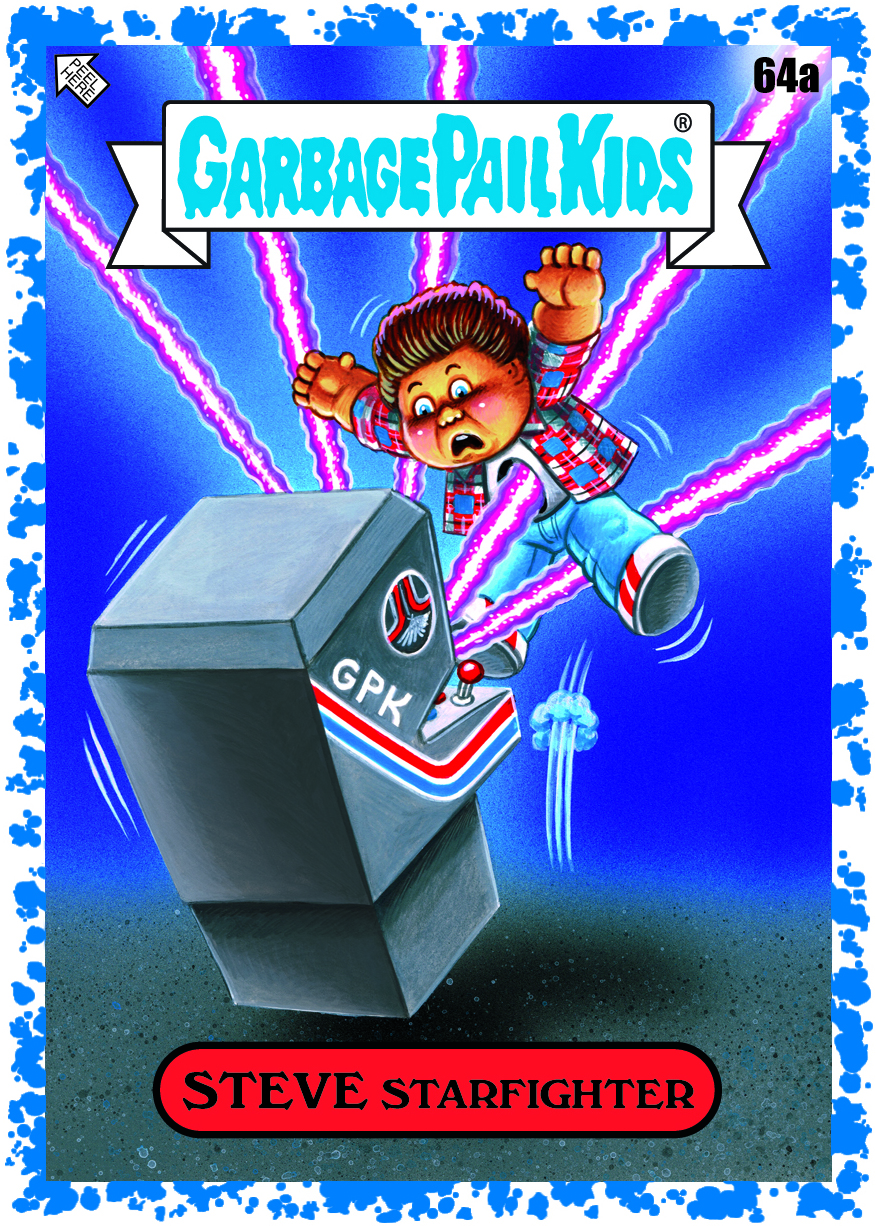This is a detailed illustration of a Garbage Pail Kids trading card titled "Steve Starfighter," numbered 64A. The card features a central image of a gray arcade machine, prominently tilted towards the left, with red, white, and blue stripes adorning its sides, and the letters "GTK" displayed on it. Emanating from the arcade machine are laser beams, one of which is striking a boy with brown hair, who is depicted mid-jump with raised hands, as if reacting to being hit. Above this chaotic scene, the text "Garbage Pail Kids" is boldly displayed, while the bottom of the card reads "Steve Starfighter." The color palette includes shades of purple, white, gray, red, blue, black, tan, and brown, creating a vibrant and eye-catching composition that nostalgically echoes the style of 1980s and early 1990s arcade game covers or comic books.